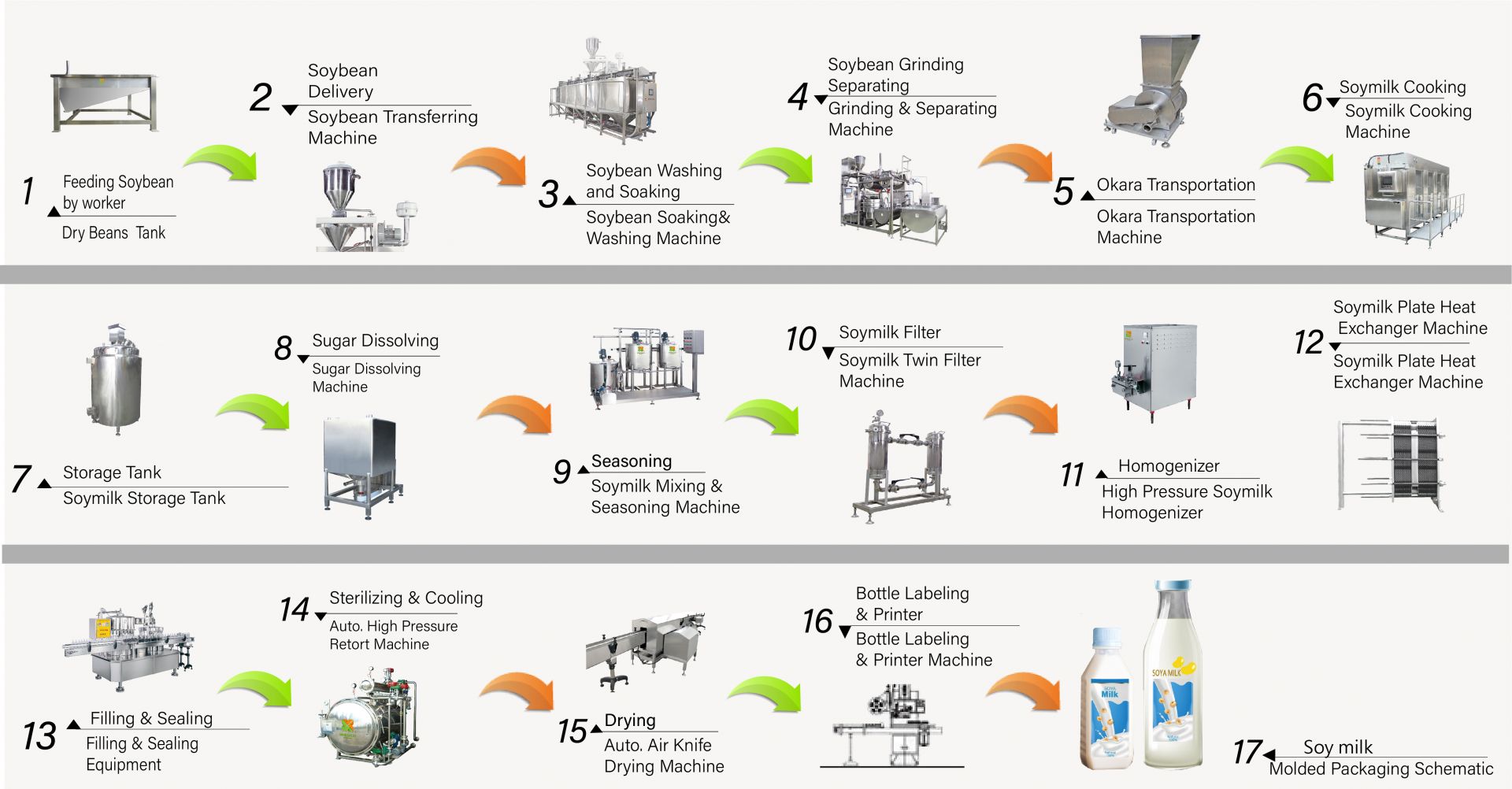**Detailed Caption:**

This is an intricately illustrated 16-step diagram that meticulously depicts the entire process of harvesting and processing soybeans into soy milk. The diagram is laid out horizontally on a white page, which is divided into three distinct tiers by two subtle gray bars. 

- In the first tier, which comprises steps one through six, the process starts with feeding soybeans into a dry beans tank and progresses through various stages, including soaking and grinding the beans, culminating in cooking the soy milk.
  
- The second tier, depicting steps seven through twelve, details the transition from cooked soy milk entering the storage tank to the passage through a plate heat exchanger machine. 

- The third and final tier outlines steps thirteen through seventeen, illustrating the stages from filling and sealing the soy milk into packages to its final form, ready for distribution.

Each step is clearly numbered and visually represented, providing a comprehensive view of the soy milk production process from raw soybeans to packaged product.